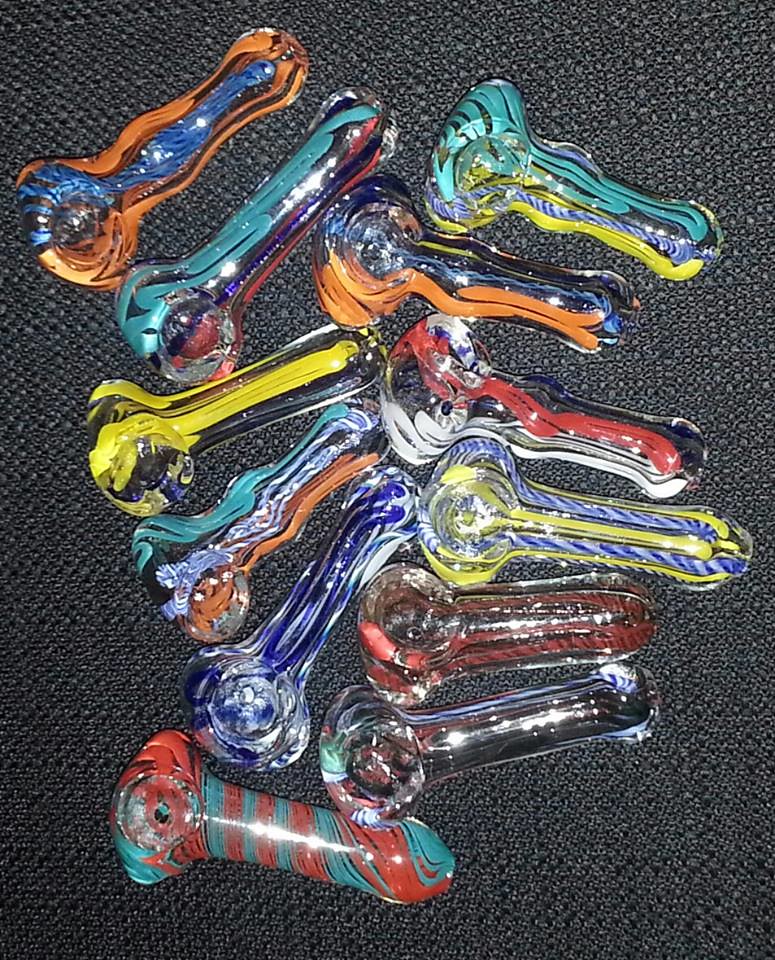This image features a collection of twelve hand-blown glass pipes, commonly used for smoking marijuana or tobacco. The pipes are arranged on a dark gray, rough-textured background that resembles woven carpet or a placemat. Each pipe is uniquely colorful, showcasing a variety of intricate designs and color combinations. For instance, the top two pipes are positioned diagonally from bottom left to top; one is orange with blue in the center, and the other is teal with red accents. On the right-hand side, additional pipes display patterns like teal and yellow, black and orange stripes, red and white, blue and yellow stripes, red and clear, and black with a teal bowl. Over to the left side, there are more pipes angled slightly, including ones that are yellow and clear, teal with light blue and orange, blue with black or white, and one almost straight across in red and teal stripes resembling a candy cane. These colorful glass pieces stand out vividly against the dark background, with some featuring a clear plastic ball at the center, which adds a distinctive touch to their design.